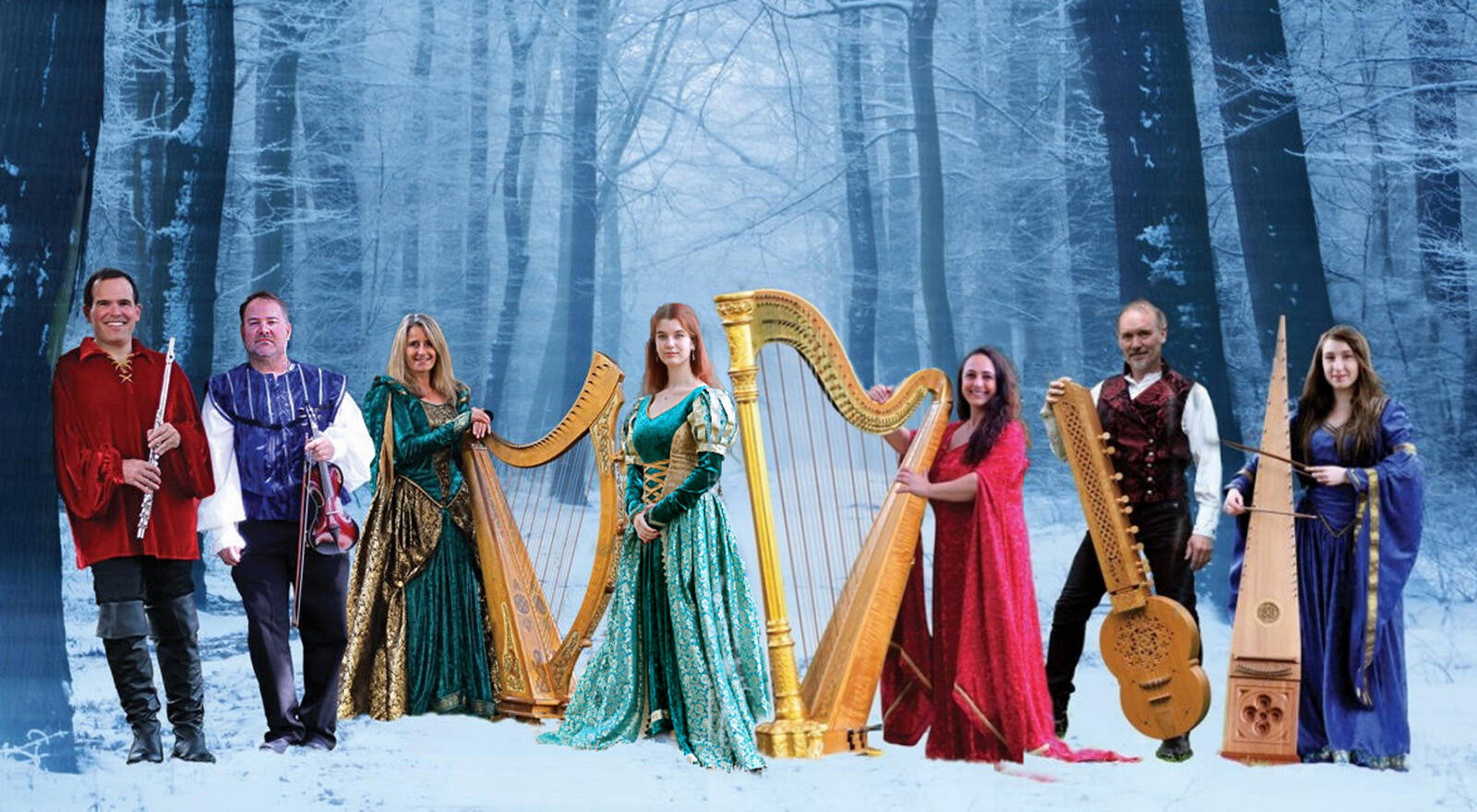The image portrays a staged scene depicting a snowy forest with tall, slim trees blanketed in snow. The background appears either artificially created or set against a green screen due to the unnatural appearance of the setting. In the foreground, a group of people dressed in elaborate, Victorian-era and Celtic folk-inspired costumes stand in the snow. The men wear flowy tops, blouses, suits, and vests, while the women don long, flowing dresses in various colors, including green and red. All of them hold vintage-looking musical instruments, with some of the men holding flutes, horns, and possibly an ancient guitar with a thick neck, and the women carrying harps and other unidentified, old-fashioned instruments. The array suggests a band, perhaps performing Celtic or classical music in this whimsically recreated, snowy landscape.